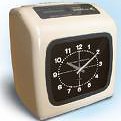The image depicts a small, squarish, and bulky device, likely a time clock, rather than a conventional alarm clock. The device, tan or off-white in color, appears to be constructed from either metal or shiny plastic. Prominently featured on its face is a black clock with white numerals and hands indicating the time as approximately 10:10. Adding to its distinct appearance, the front face also includes an inner gray circle encircling the numbers and the clock hands. Located at the top of the device is a dark grey or black rectangular section, potentially the slot for inserting time cards. Despite the image's small size, the clock's robust and boxy structure distinguishes it as a specialized timekeeping tool rather than a standard bedside alarm clock.